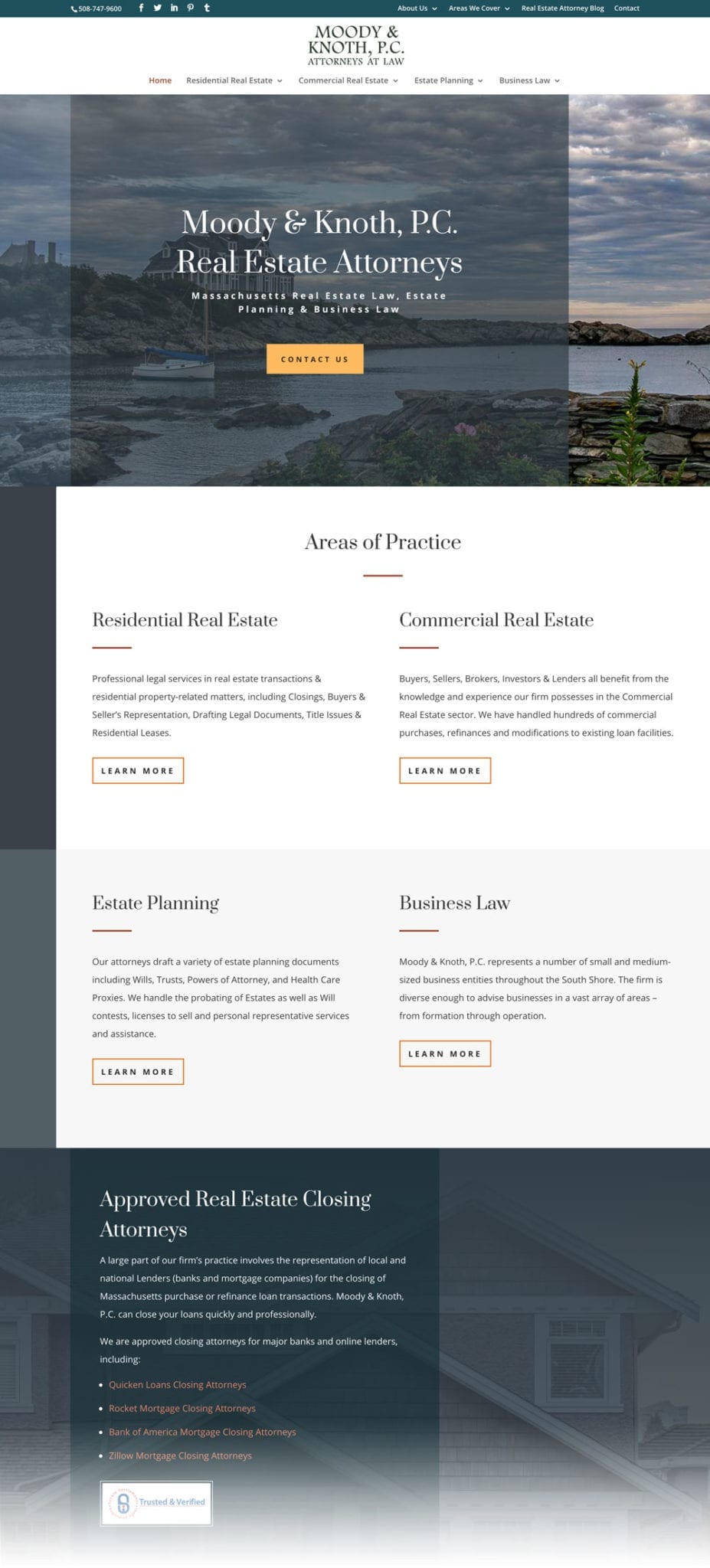Screenshot of the website for Moody and Knoth PC Attorney at Law, a Massachusetts-based real estate law firm named after its founders, the self-made attorneys Mr. Moody and Mr. Knoth. The website highlights their areas of practice, specifically residential real estate, commercial real estate, business law, and estate planning. Moody and Knoth are approved closing attorneys for prominent lenders including Quicken Loans, Rocket Mortgage, Bank of America, and Zillow. The background of the website features images of newly built houses, residential estates, and a serene stream running beside one of the new properties, emphasizing their focus on real estate law.